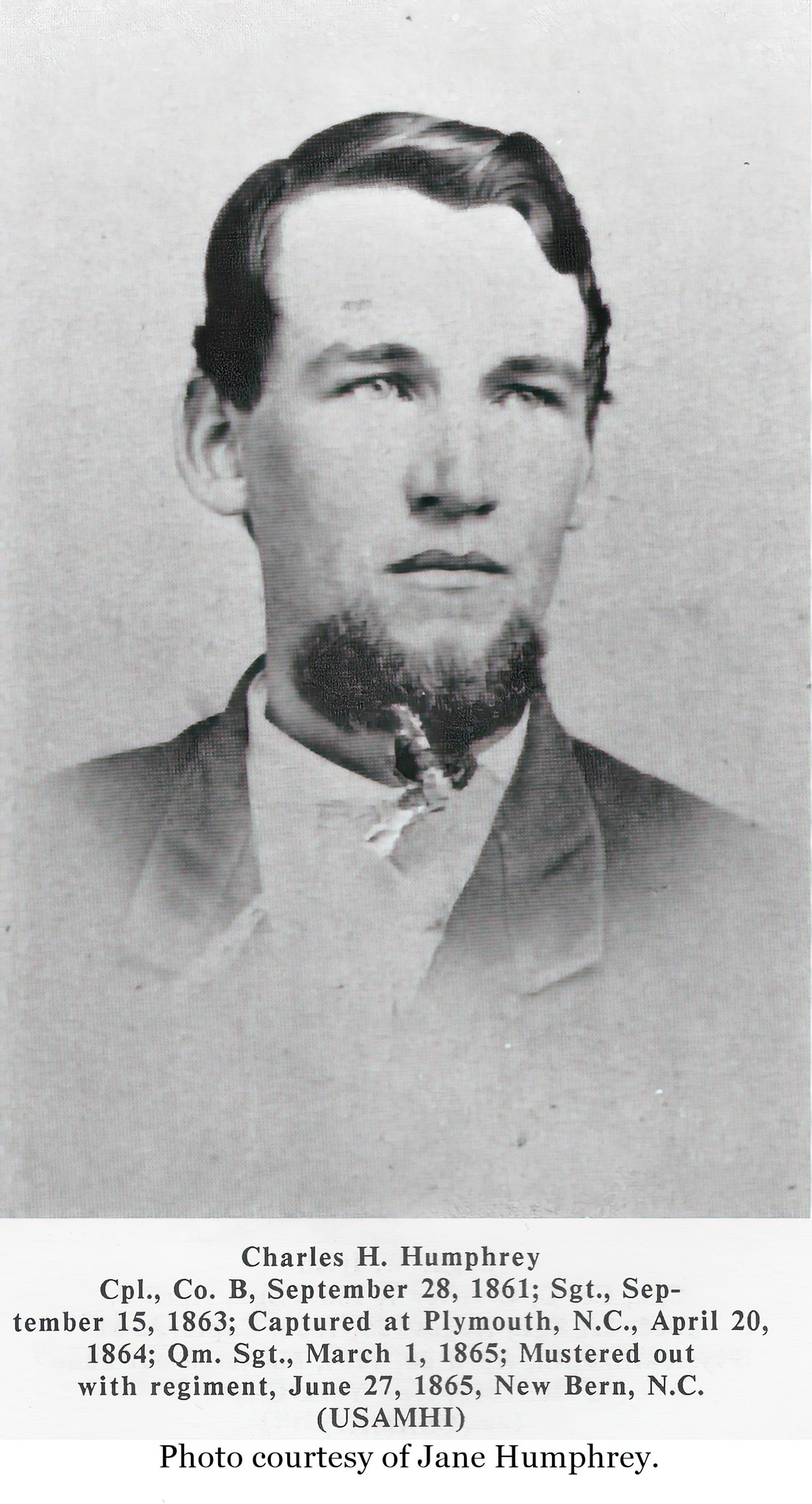This is a very old, 19th-century black-and-white photograph depicting a white man in his 30s or middle age with a neatly combed and right-parted hair. He sports a neck beard and gazes stoically to the right. The photograph is worn, showing signs of age, including a hole where the beard is. Below the photograph, an inscription reads: "Charles H. Humphrey, Corporal, Company B, September 28, 1861. Sergeant, September 15, 1863. Captured at Plymouth, North Carolina, April 20, 1864. Quartermaster Sergeant, March 1, 1865. Mustered out with regiment June 27, 1865. New Bern, North Carolina, USA MH-1." The photo is noted to be courtesy of Jane Humphrey.